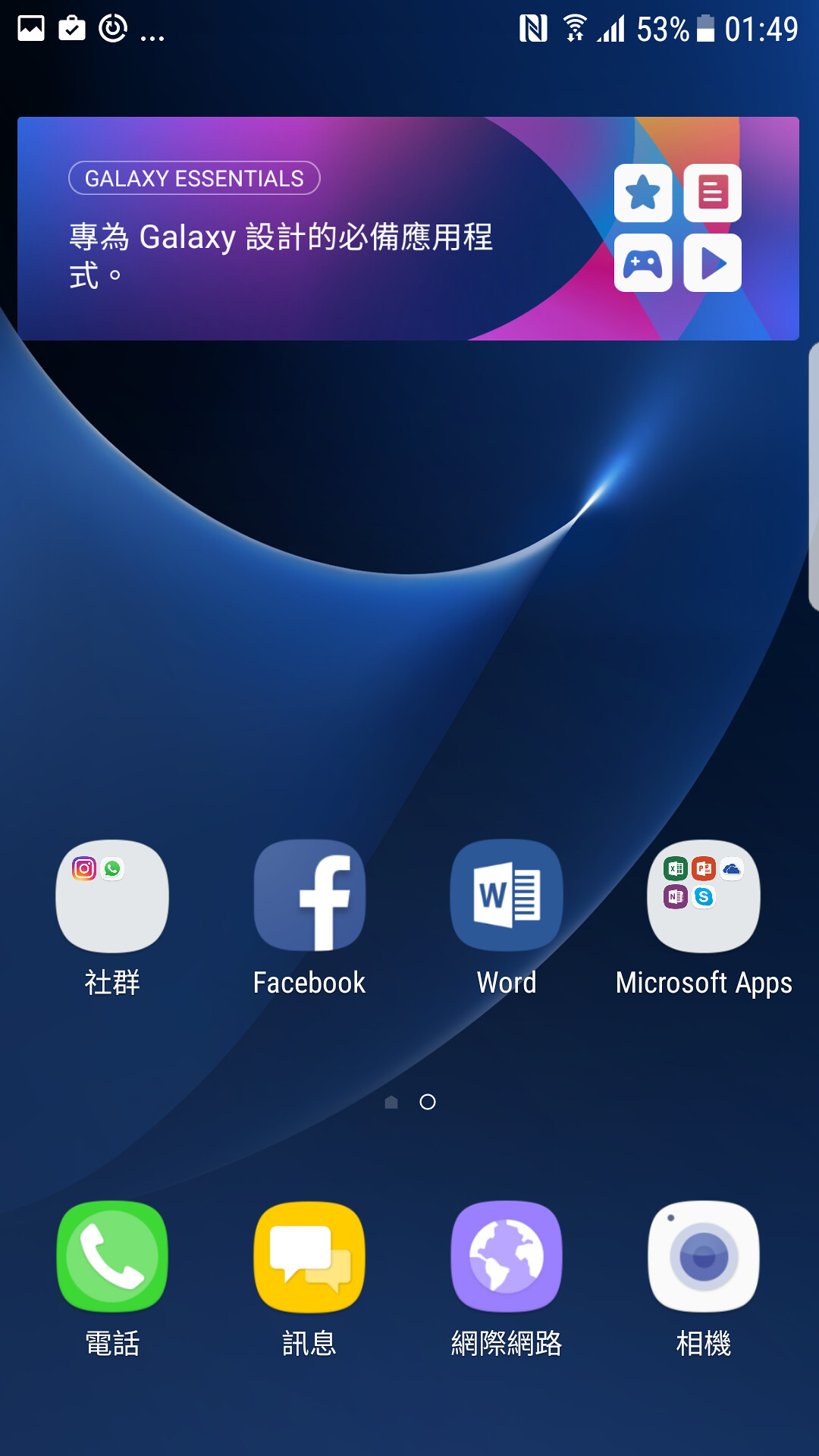A detailed screenshot of a Galaxy smartphone screen. At the top, a series of icons are visible: a mountain icon indicating photos, a check mark with a briefcase, a circular icon followed by three dots, an "N" symbol, Wi-Fi signal, cellular signal with four bars, battery percentage at 53%, battery icon, and the current time displayed as 1:49. Below these icons, there is a banner labeled "Galaxy Essentials" accompanied by Chinese characters and "Galaxy." To the right of this banner are four additional icons. The background of the screen is dark blue with a black hole-like motif, blending shades of blue and black. The app icons featured on this screen include an app with Chinese characters, Facebook, Microsoft Word, Microsoft Apps, a green phone icon indicating the phone app, a text messaging app, the camera app, a web browser app, and several others. All app labels are depicted with Chinese characters underneath.